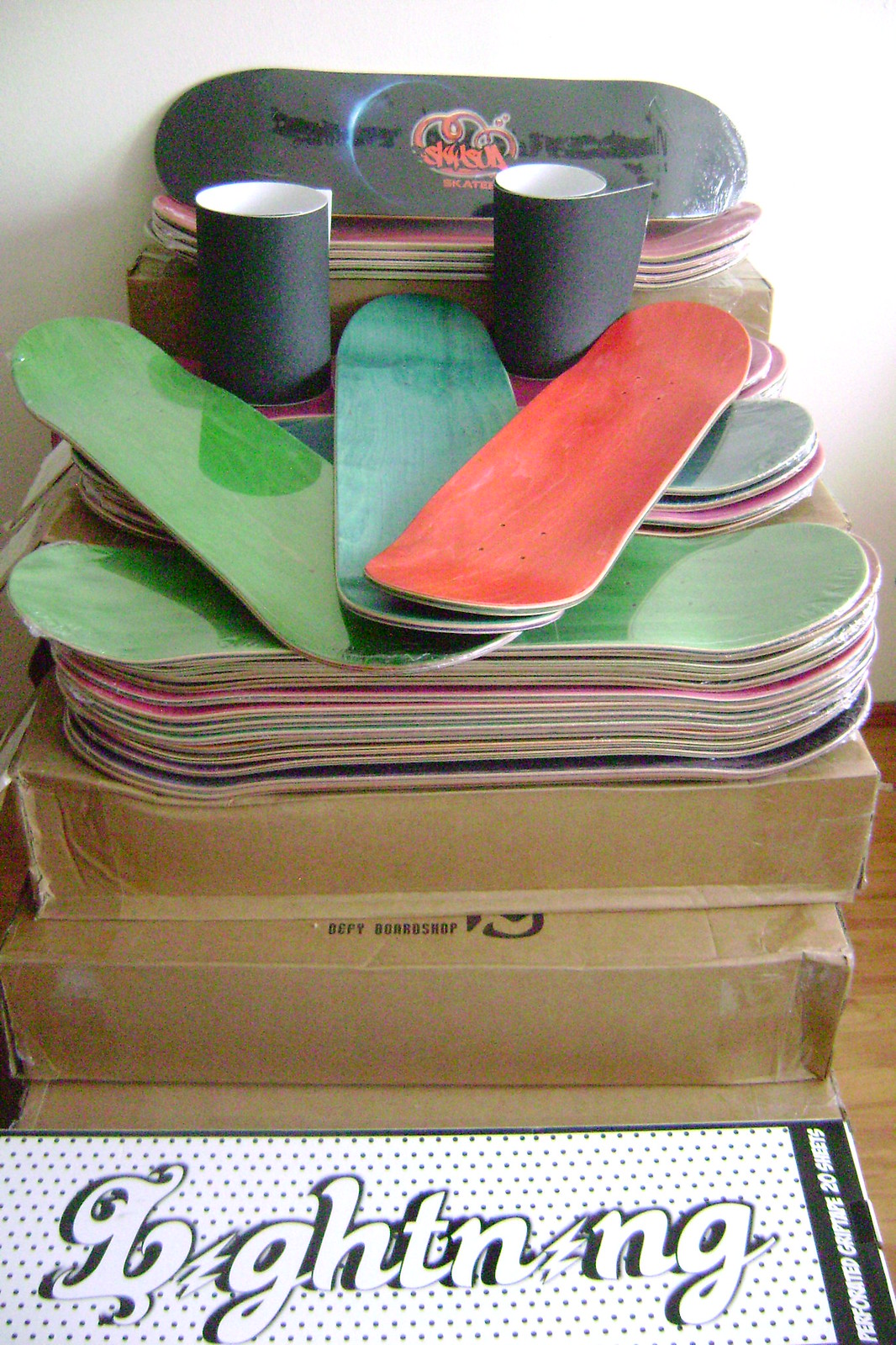This image captures a detailed side view of multiple stacks of skateboard decks without wheels. The skateboards are symmetrically organized in four vertical stacks, varying in colors such as green, blue, red, and gray. Alongside the columns, three decks are arranged in a trident shape on top, with the colors green to the left, blue in the middle, and red to the right. They are positioned atop two brown cardboard boxes, slightly offset to reveal parts of both. The scene is set on a wooden floor, partially visible at the bottom of the image. Toward the front, a white mat with alternating black and white borders and black polka dots is prominently displayed. It features a stylized text "Lightning," with the 'i's replaced by lightning bolts, and additional smaller text mentioning "perforated or grip line 20 sheets." Above the skateboard stacks, there are two black rolled-up sheets, likely grip tape for the skateboards. In the background, a black skateboard leans against a white wall, adorned with a red design and graffiti-styled text "skater." The detailed composition and organized layout of the skateboards present a visually appealing arrangement.